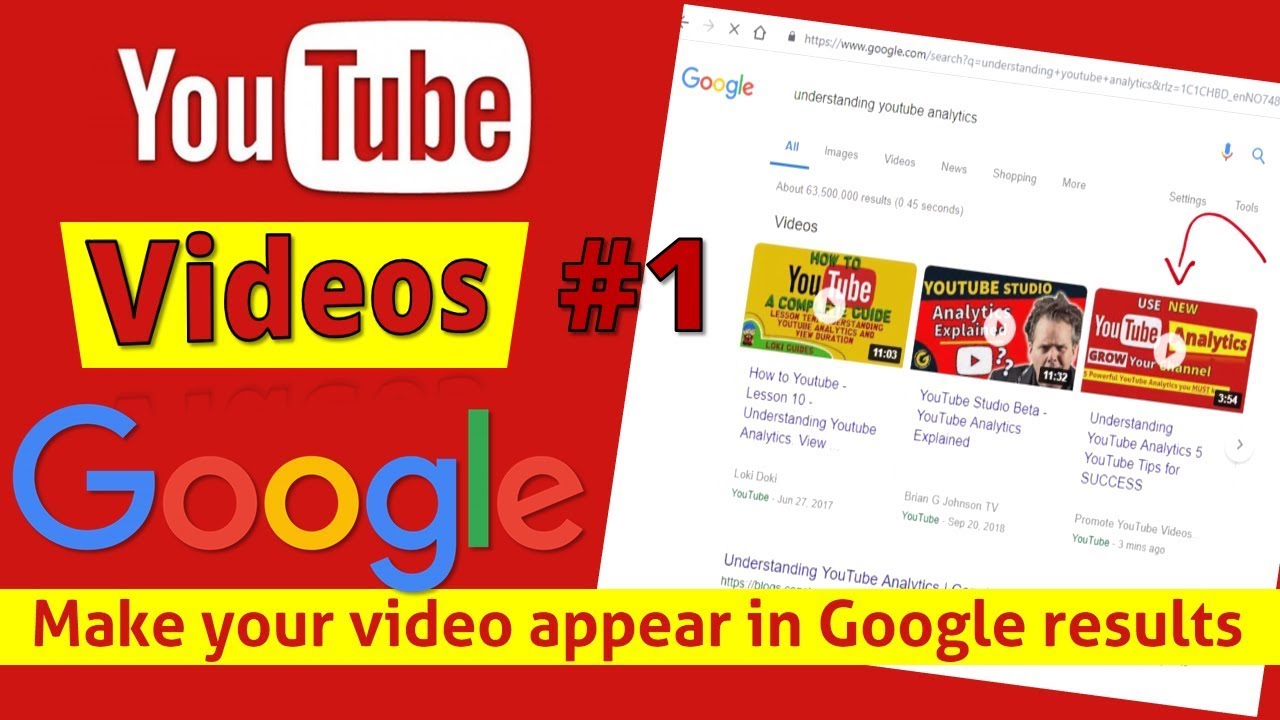The image is a vibrant, colorful advertisement set against a bold red background. At the top, the iconic YouTube logo is prominently displayed, with "You" in white and "Tube" in blue, enclosed within a white TV frame. Below it, a yellow box with red text reads "VIDEOS," accompanied by a red hashtag and the number "1."

Adjacent to this, the Google logo is featured, with its letters in their trademark colors: "G" in blue, "O" in red, "O" in yellow, "G" in blue, "L" in green, and "E" in red. A yellow bar runs horizontally across the image, displaying the red text, "Make your video appear in Google results."

On the right-hand side of the screen, there is a angled screenshot of a Google search page with a URL that reads: "www.google.com/search?q=understanding+YouTube+analytics&RLZ=1C1CHBD_EN0748". Below this, it says "Next" followed by the Google logo and "Understanding YouTube Analytics."

The screenshot displays three video results:
1. "Understanding YouTube Analytics View - YouTube Studio Beta - YouTube Analytics Explained" by "LokiDoki," uploaded on June 27, 2017.
2. "Understanding YouTube Analytics 5 - YouTube Tips for Success" by "Brian G Johnson TV," uploaded on September 20, 2018.
3. "Promote YouTube Videos" by "Promote YouTube Videos," uploaded three minutes ago.

The layout and typography guide the viewer's eye through the promotional material, emphasizing the ease of making videos appear in Google search results and offering insights into understanding YouTube analytics.